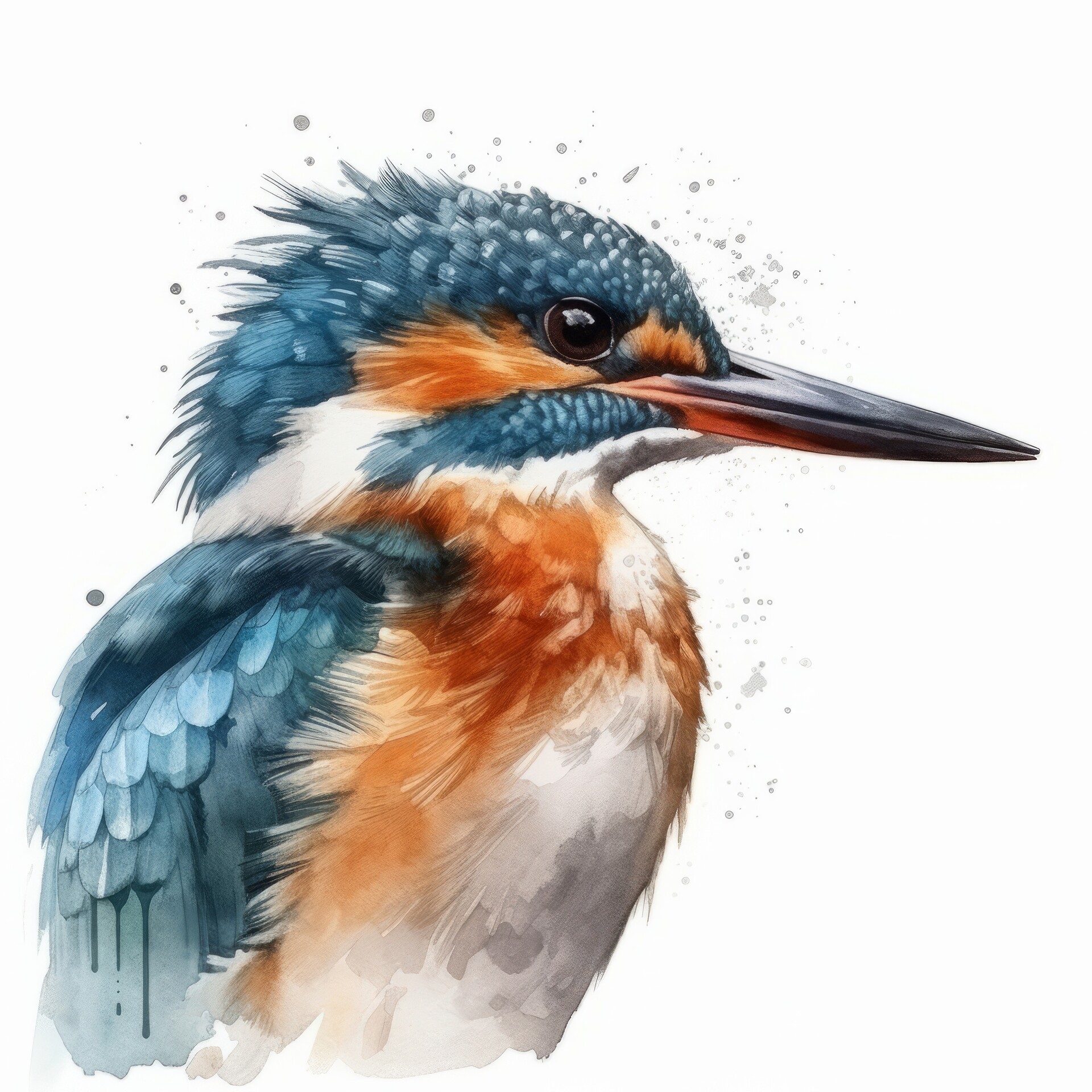This image depicts a computer-generated, cartoon-style bird with vibrant, watercolor-like features set against a white background. The bird, captured in a close-up profile view, exhibits a striking blend of colors: its head, back, and wings are adorned with a soft blue hue that edges into a grayish tone, while its breast feathers are predominantly white. Accents of burnt orange feathers embellish its face beneath its dark eye and near the chest. The bird's long, slender beak transitions from a mix of light red and orange at the tip to a dark gray, almost black, further down. Surrounding the bird are gray and blue shadowy splatters, resembling droplets of water, adding dynamic motion to the composition. The harmonious interplay of the bird's colors and the delicate details make the image visually appealing.